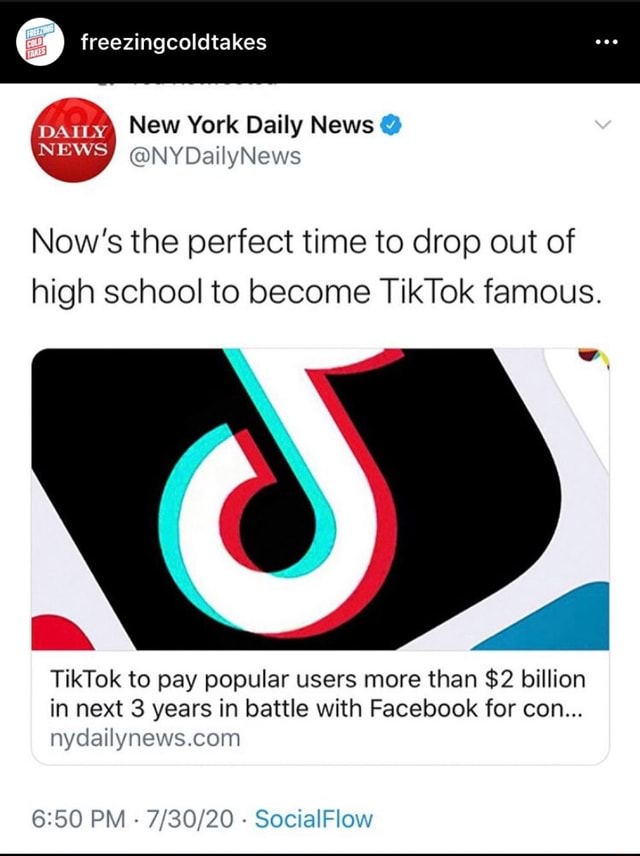This image appears to be a screenshot from Twitter. The top portion of the screenshot has a black background with a white circle in the upper left corner featuring small, indistinguishable text. Next to this circle, the words "Freezing Cold Takes" are prominently displayed in white text. To the right of this text, three white dots are arranged vertically.

The main section of the image has a white background. A red circle containing the text "Daily News" in white is positioned to the left of the text "New York Daily News," which is written in black. To the right of this text, a blue circle with a white checkmark signifies that the account is verified. Beneath this, the Twitter handle "@NYDailyNews" is displayed.

The tweet itself reads: "Now's the perfect time to drop out of school to become TikTok famous." Accompanying this text is the TikTok logo, followed by the message: "TikTok to pay popular users more than $2 billion in the next three years to battle with Facebook for CON..." The tweet's timestamp is 6:50 PM on July 30, 2020.

At the bottom of the image, 'social flow' is indicated, followed by a black line.